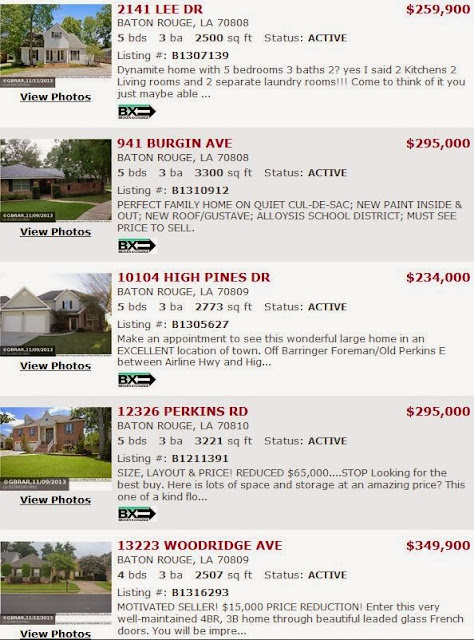The image displays a collection of five housing listings for sale. For each listing, a photograph is shown on the left side with a clickable link that reads "View Photos" to access additional images. The listings prominently feature the address and price in large, red lettering, with the addresses on the left and prices on the upper right corner.

1. The top listing showcases a white-painted, two-story house located at 2141 Lee Drive, Baton Rouge, Louisiana, 70808. It is priced at $259,900. This residence boasts five bedrooms, three bathrooms, 2,250 square feet of living space, and it is currently active on the market.
2. The second listing features a single-story brick home at 941 Virgin Avenue, Baton Rouge, Louisiana, 70808, listed for $295,000. Specific details regarding the number of beds, baths, and square footage are also provided.
3. The third property is a two-story white house with a two-car garage, situated at 10104 High Pines Drive, Baton Rouge, Louisiana, 70809, with an asking price of $234,000.
4. The fourth listing presents a two-story brick home located at 12326 Perkins Road, Baton Rouge, Louisiana, 70810, available for $295,000.
5. The bottom listing displays a single-story home with a spacious yard, set at 13223 Woodridge Avenue, Baton Rouge, Louisiana, 70809, priced at $349,900.

Each listing further includes detailed information about the number of beds, baths, square footage, status, and the unique listing number, along with brief descriptions of the properties.